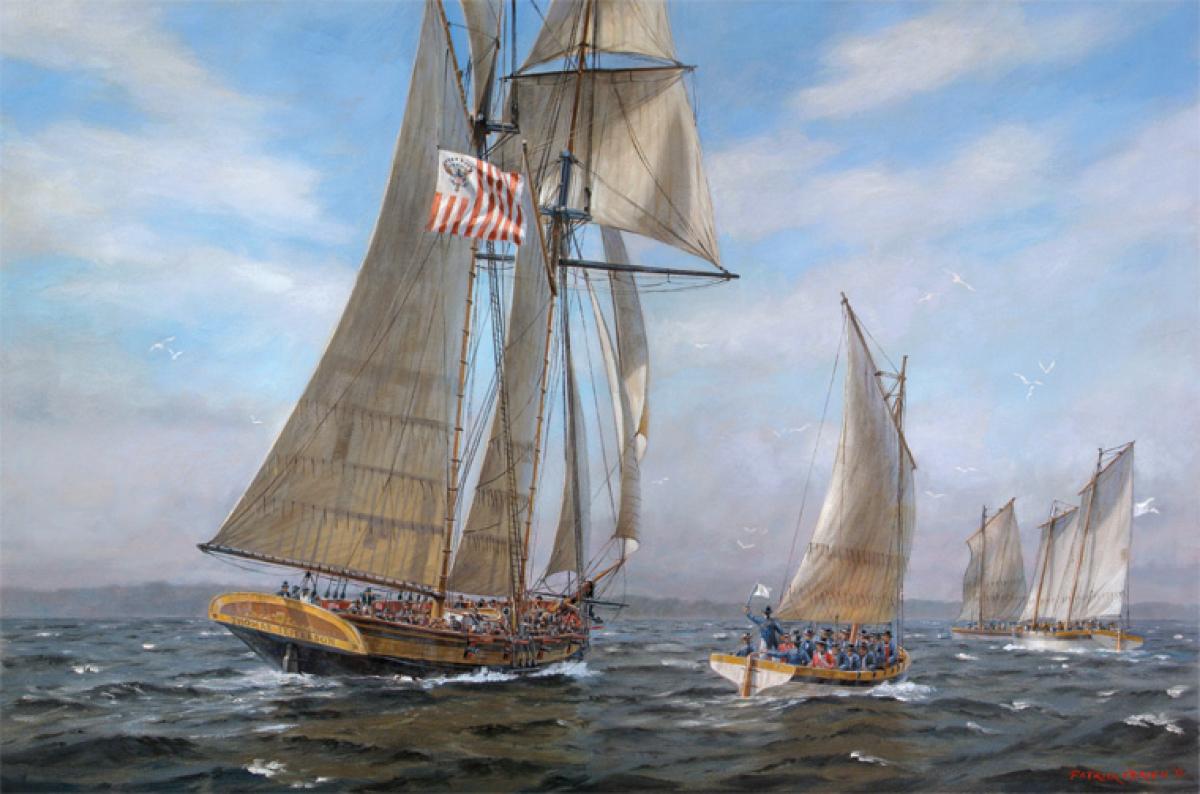The image captures a serene yet vibrant maritime scene, possibly a regatta, featuring multiple sailboats against a vast blue sky with puffy white and gray clouds dominating about 70% of the background. The dark, choppy water below reflects a lively seascape with visible ripples and waves. The primary focus is a large sailboat with multiple open sails in shades of white and off-white. This prominent ship, detailed with a brown and black hull, hosts numerous indistinguishably small figures onboard. A prominent flag with red and white stripes and an emblem, perhaps an eagle, waves from one of its beams.

Nearby, a smaller sailboat, white with a brown trim and a hint of yellow, also hoists its white sails proudly. The people on this boat, many in red and blue coats, crowd the vessel, with one figure in a blue coat waving a white flag. In the background, two more sailboats with white sails drift along, their lighter-colored hulls barely discernible. The entire scene is an artist's meticulously detailed painting, signed in red at the bottom right corner, though the signature is too small to read. Subtle mountain-like forms rise in the far distance, adding depth to this engaging nautical tableau.